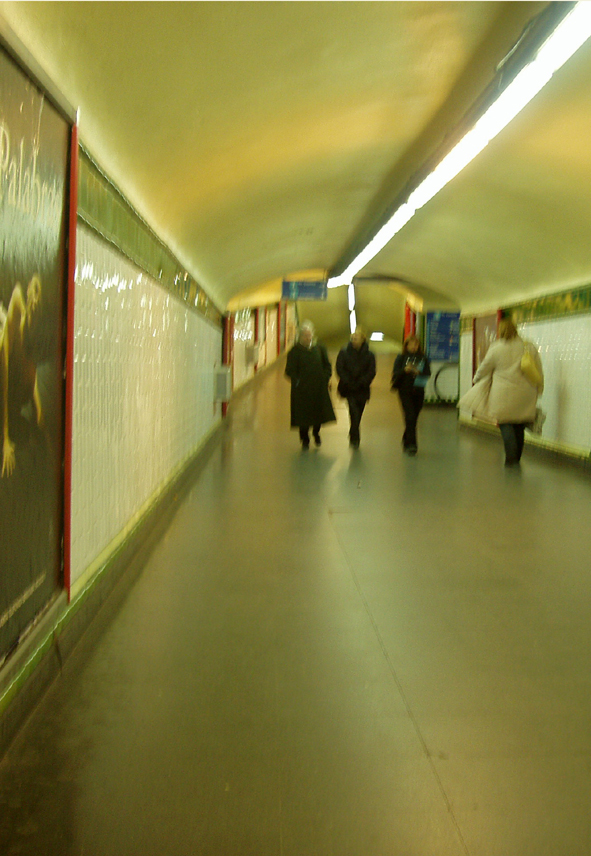In the image, a wide hallway with a yellowish tint can be seen. Although the photograph is blurry, there appear to be three women walking in one direction and one woman walking in the opposite direction. The walls of the hallway are predominantly white and feature a decorative border at the top. The flooring seems to be made of large, white tiles, adding to the overall brightness of the space. The exact location or type of building is unclear due to the blurriness of the image.